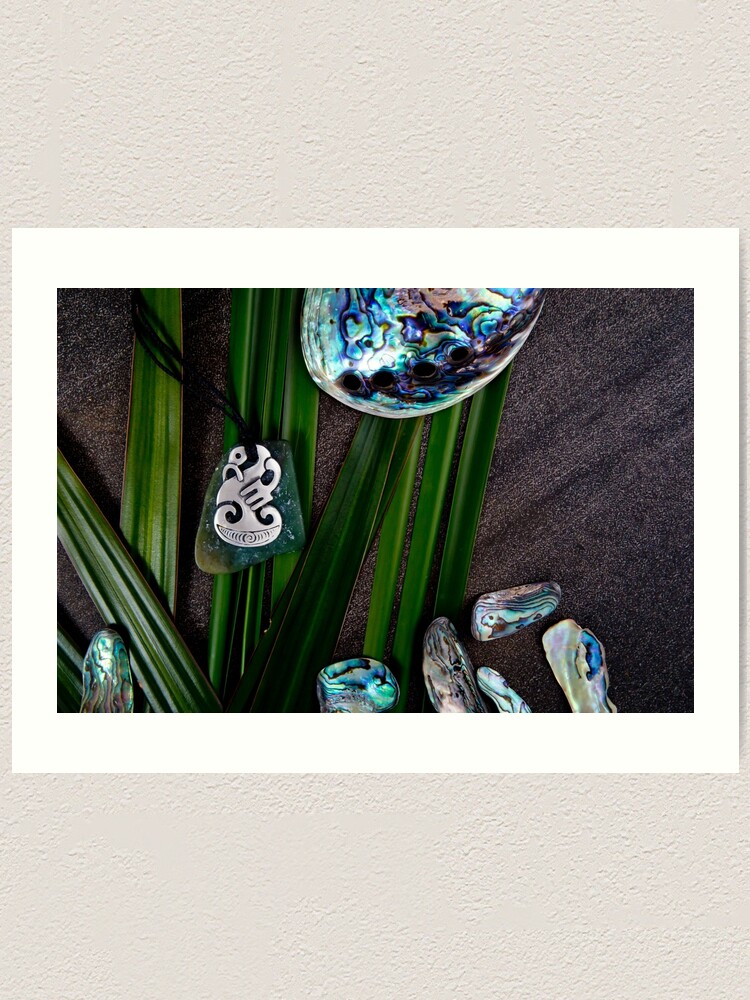The image depicts an intricately styled product photograph featuring a piece of artwork. At the forefront, there is a silver medallion with a curved shape, attached to a black cord. This medallion is centrally positioned among an arrangement of long, dark green foliage, bearing a resemblance to aloe leaves with distinctive lines on their surfaces. Surrounding the medallion are six iridescent stones showcasing vibrant and reflective patterns in hues of turquoise blue, aqua blue, silver, and black. These stones possess a captivating metallic sheen, with one larger stone prominently placed near the top of the photograph. The entire composition rests on a dark, presumably charcoal black background, enhancing the vividness of the stones and foliage. An additional detail includes a white border framing the central image, set against a light gray or beige textured backdrop, giving the entire piece a polished and artistic presentation.